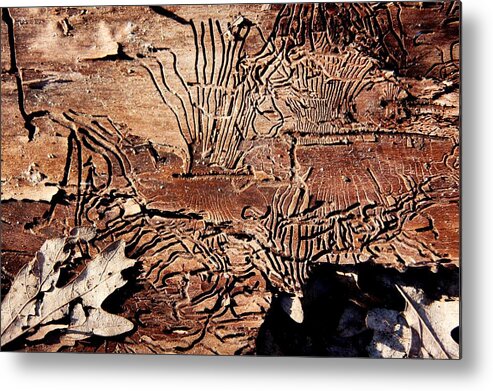This photograph captures a close-up of a piece of wood ravaged by termite or beetle infestation, highlighting an intricate network of tunnels and lines that zigzag across its surface. The image, in landscape orientation, depicts the wood with varying shades of light and dark brown, showcasing the damage left by the insects. The most prominent feature is a dense cluster of dark termite trails in the center, resembling multi-stemmed pieces of wheat. The wood appears flat, potentially bark, and is likely laying on the ground, possibly supported by a brick visible in the lower right corner. The bottom left corner of the image features a large, decaying brown oak leaf, brittle and falling apart. Additionally, the lower right section with a chunk missing reveals more leaves beneath the wood. The overall composition merges the earthy tones of the insect-eaten wood with the red and cream hues of its surroundings, giving the photograph an artistic feel, almost like a metal print artwork.